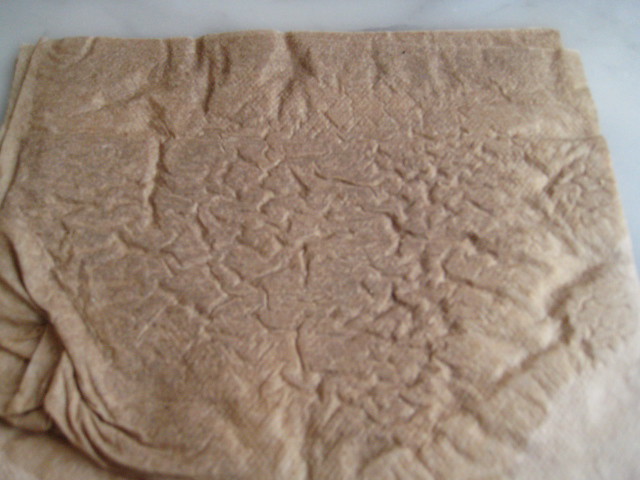The image depicts a rectangular photograph showing a brown, soggy, and folded item that resembles napkins or dough, with a textured surface covered in myriad lines, creases, and crumples. The item occupies the majority of the image and appears somewhat rectangular but with irregular, folded edges, especially visible in the lower left-hand corner where it's bunched up. The left side of the item is slightly pulled away to reveal another similar item underneath. The right-hand side of the item has lightened, possibly due to drying, and appears almost white. The background of the image is a light gray, possibly a stone countertop.